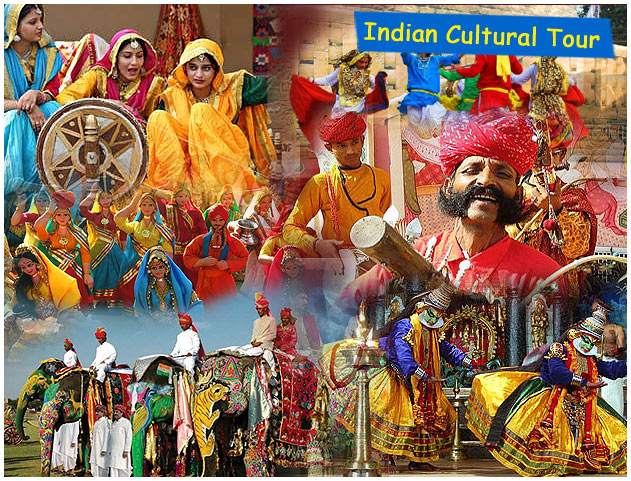The image is a vibrant photo montage showcasing a celebration during an "Indian Cultural Tour," prominently labeled at the top in yellow Comic Sans font against a bright blue background. The participants, all of Indian descent, are adorned in strikingly colorful traditional clothing. On the top left, three women are seen in eye-catching saris in yellow, green, pink, and blue. Centrally and at the top, a woman captures attention as she dances gracefully. To the middle left, a group of people wear brightly colored costumes and elaborate headdresses. On the top right, a man in a red turban and outfit plays with a tube-like instrument. At the bottom of the image, both men and women ride on richly decorated elephants. Also depicted are performers in gold dresses bowing towards the stage. This diverse collage encapsulates the rich tapestry of Indian cultural attire and festivities.